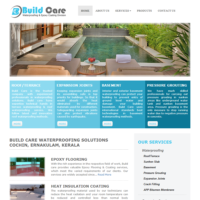A small, highly detailed screenshot of a website. The top of the page features the name of the website, which appears to say "Build Core" or possibly "Build Care," with "Build" prominently displayed in blue and "Care" or "Core" in black. The logo is positioned to the left of this text. 

To the right, there are five navigation tabs. The first tab is highlighted with a pale gray border, while the remaining four tabs are simply labeled without any additional outline.

Directly below, the main content begins with a large photograph spanning the width of the screen. It portrays a lush, outdoor poolside setting featuring a rectangular pool surrounded by chaise lounges. Brown-framed doors, likely leading to a pool house or main house, are visible in the background, along with abundant vegetation. The image appears to be an illustration rather than a real photograph.

Beneath the poolside scene are four colored squares, each containing white text and a white button in the bottom left corner. The first square is light blue, and the subsequent squares form an ombre effect that starts with light blue on the left and transitions to dark teal blue on the right. The colors are, in order from left to right: light blue, slightly darker aqua blue, turquoise light blue, and teal.

Further down, there is a text section under the heading "Build Care Waterproofing Solutions" followed by a brief, unreadable description. Below this section, there are two thumbnail photographs accompanied by descriptions to their right.

The final portion of the screenshot shows a pale gray, vertically oriented rectangle labeled "Our Services" in blue text. This section lists nine different services in black text, but the font is too small to discern the specifics.